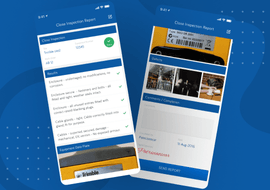A screenshot depicts a blue background adorned with a grid of white dots in the lower left and upper right corners. Nestled within this backdrop are two slightly diagonal smartphone screenshots. The left phone slants a bit to the left while overlapping slightly with the bottom right corner of the right phone, which is angled slightly to the right. Both screenshots are rather small, making it difficult to pinpoint the exact websites displayed, though both feature blue and white color schemes.

The left screenshot prominently showcases three blue bars interspersed with white sections containing black text. At the very bottom of this screenshot, a yellow and silver item is vaguely visible, potentially extending into the top segment of the left screenshot. Below this section, three images are displayed in a row, followed by a white space, and ultimately, a blue button at the bottom.